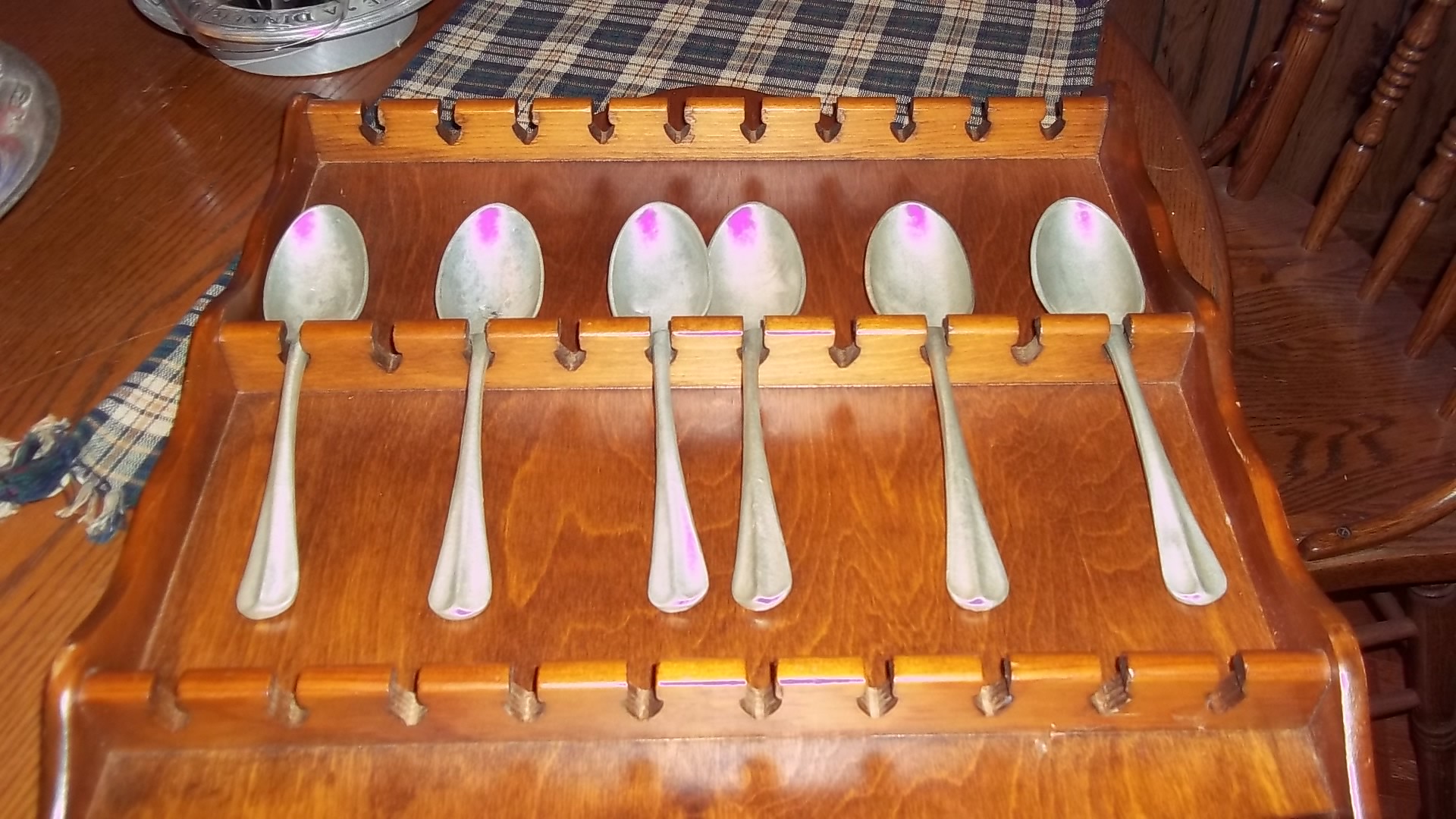The photograph features a vintage wooden display case resting on a slightly lighter colored brown wooden table. The display case, designed to hold utensils, contains six antiquated silver spoons, each adorned with a slight magenta or purplish tint at the tips. Notably, the first four spoons have this coloration on the left side of their tips, while the last two display it on the right. Among them, the third spoon from the left exhibits some of this coloration on its handle, and a few others show faint traces of it as well. The display case is structured with several notches to support utensils, featuring three visible rows, each capable of holding 10 spoons, though currently housing only six. The case itself is made of dark wood, complementing the table’s hue. A blue and white plaid placemat lies beneath the rack, with the corner of another placemat peeking into the frame from the lower left. Two indistinct circular objects, one appearing plastic and the other metallic, are partially visible in the upper left of the image. Additionally, a wooden chair with a visible seat and back spindles is positioned to the right, and a wooden paneled wall is detectable in the background on the right side of the photograph.